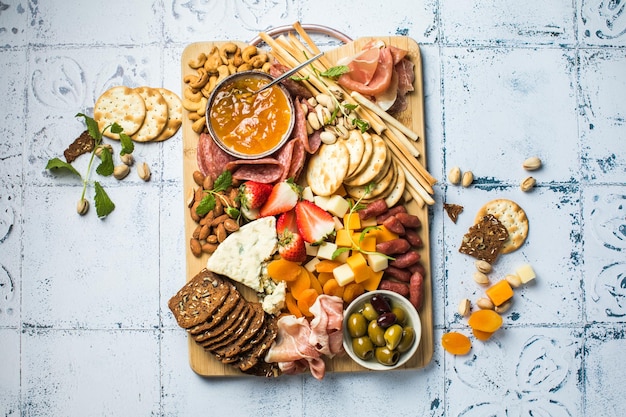This photograph captures a detailed arrangement of a charcuterie board set against a light blue tile background with decorative patterns. The wooden charcuterie board is brimming with a variety of delectable items, some even spilling onto the tile. Centered on the board is a silver bowl containing apricot jam with a spoon, bordered by elegantly folded salami and nestled almonds. To the board's left, there are three wheat crackers accompanied by five pistachios and a mint leaf. Nearby, cashews are scattered, adding to the nutty assortment. 

Arrayed on the board are halves and whole strawberries, slices of prosciutto, and a mix of cheeses, including a large chunk of blue cheese or possibly gorgonzola, as well as cubed cheddar and white cheese. Long and circular crackers are positioned strategically, while a piece of toasted bread with embedded nuts provides texture. Green olives and two black Kalamata olives rest in a white bowl next to more prosciutto and additional pistachios. Above the olives, small sausages and apricots add to the intricate display. Scattered around the board and onto the tile, one can find square cubes of cheese, extra crackers, and microgreens delicately sprinkled over the selection, enhancing the visual feast.